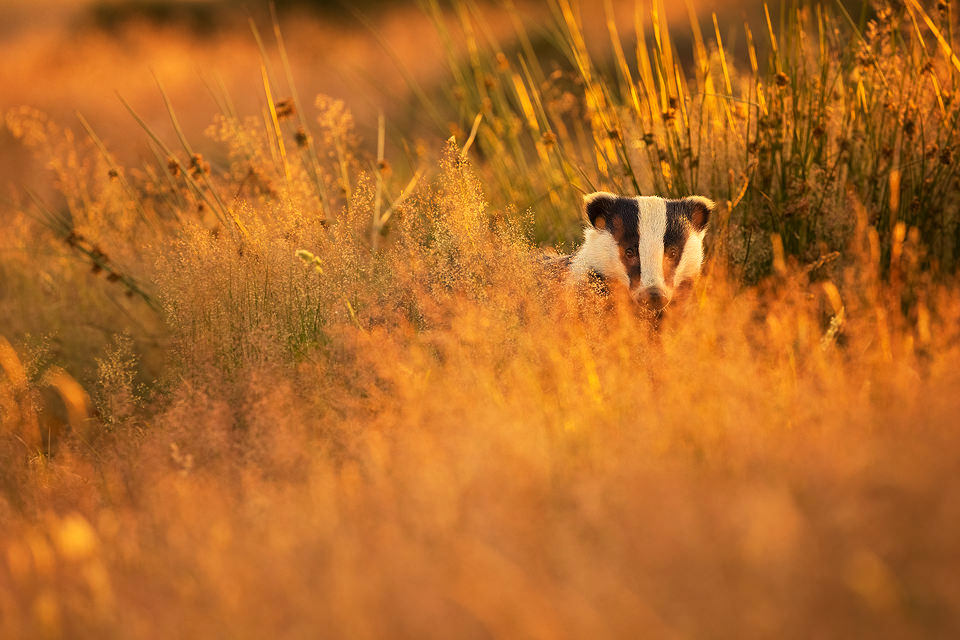In a sunlit field, a medium-sized dog stands with its head facing the camera. The surrounding field features a mix of tall grasses, which appear in varying shades of green, yellow, and brown, slightly blurred both in the foreground and background. The sunlight, coming from the right, enhances the warm tones of the scene, giving it a bright, almost golden hue. Situated slightly to the right of the image's center, the dog's head and upper shoulders are visible above the grass.  Its head boasts a striking contrast: dark and light brown fur forms a symmetrical pattern on either side of a thick white streak that runs from the top of its head down to its nose. The dog's ears are small and slightly flopped. The lower part of its face and body are white, creating a clear distinction against the sunlit field.